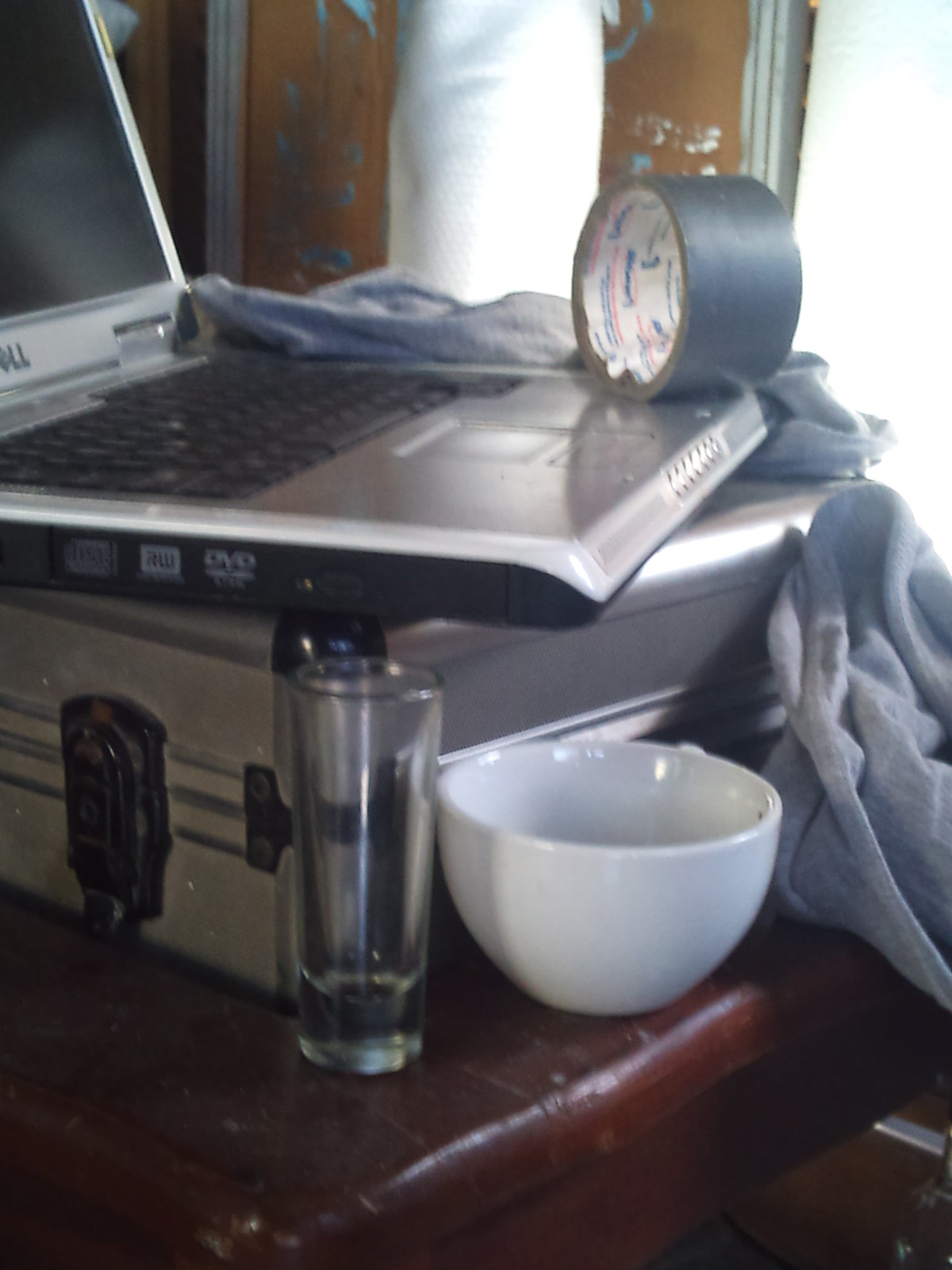A silver laptop partially displaying its screen and black keyboard rests atop a silver briefcase with black latches on a dark brown wooden table. In the background, a wooden wall splattered with paint adds an artistic touch to the scene. A transparent drinking glass and a white bowl are placed beside the briefcase on the table. A bundled-up piece of gray clothing lies next to the briefcase. A roll of gray duct tape stands upright on the laptop, revealing its white inner core. The surrounding walls, predominantly white and well-lit, contrast with the wooden wall. An indistinct object, possibly a pillow, is also visible in the background.